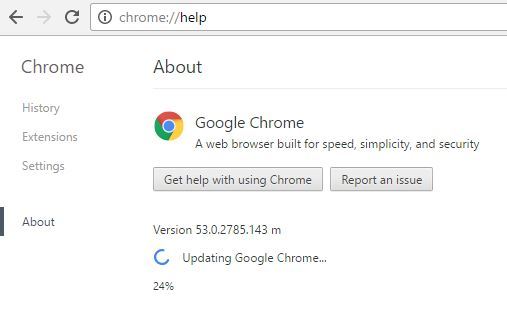The image appears to be a screenshot from a computer, specifically showcasing a Google Chrome help page. 

At the very top, we see the URL bar displaying "chrome://help" with a small eye icon enclosed in a circle next to it. The text "chrome" appears slightly lighter than the rest of the URL.

To the left of the URL bar, three navigation icons are visible: a refresh icon, a right arrow, and a left arrow.

Directly below the URL bar, on the left side, there are several menu options listed in large and small text. From top to bottom, they read:
- "Chrome" in large text
- "History" in smaller text
- "Extensions"
- "Settings"
- "About"

Next to the last option, "About," there is a small, thin black bar.

On the right side of the page, there's a larger heading that says "About." Underneath this heading, the Google Chrome icon is shown, followed by the text "Google Chrome - a web browser built for speed, simplicity, and security."

Below this description, there are two gray buttons with black text. The first button reads "Get help using Chrome" and the second says "Report an issue."

Towards the bottom of the page, in smaller text, the version of Google Chrome is shown: "Version 53.0.2785.143 m." Additionally, there is a progress bar indicating that Google Chrome is currently being updated, with the update 24% complete.